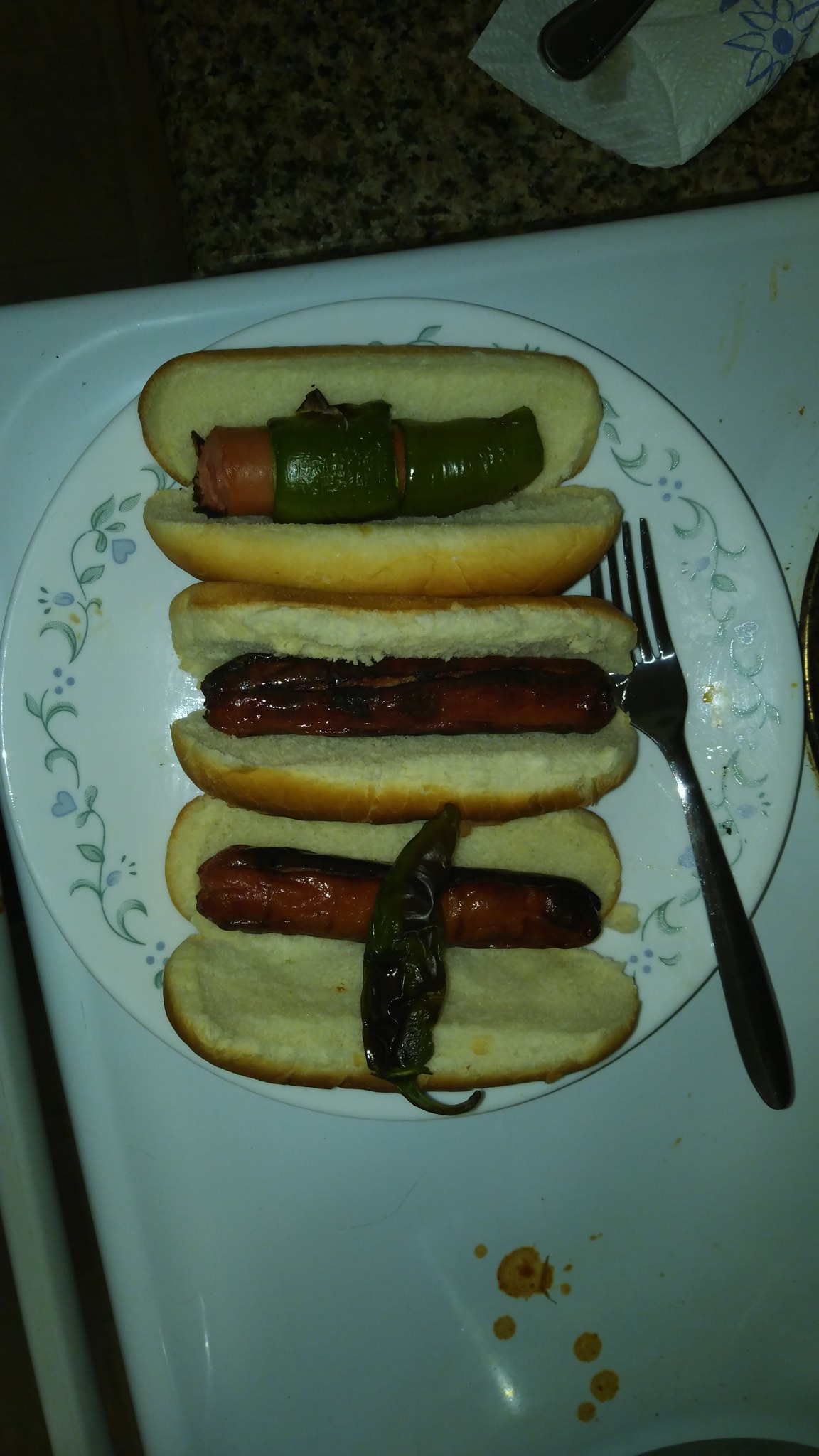The image shows a top-down view of a white plate adorned with a green vine border and small blue flowers, placed on a white tray or table. Arranged horizontally from top to bottom, the plate holds three hot dogs nestled in slightly yellowish buns, possibly due to dim lighting. 

- The top hot dog is wrapped with a grilled green pepper.
- The middle hot dog is simply barbecued without additional toppings.
- The bottom hot dog features a grilled jalapeno pepper laid perpendicularly across it.

A stainless-steel fork is positioned on the right side of the plate. Near the lower right corner of the tray, there are a couple of splotches of what appears to be tomato sauce or ketchup. In the upper right, a roll of paper towels is partially visible, along with a dark brown area that might be a tablecloth.